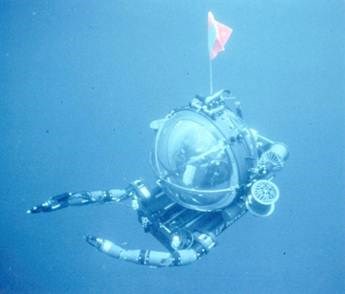This underwater photograph captures a compact, submergeable vehicle set against a blue ocean background. The centerpiece is a clear, rounded cockpit likely designed for a single occupant, although it's unclear if anyone is inside. This cockpit is affixed to a rectangular, dark-colored mechanical base that appears akin to a wooden crate. Emerging from the front of the base are two segmented robotic arms, reminiscent of crab claws, with multiple joints allowing for intricate movements and finger-like appendages at the ends. Atop the cockpit extends a small flagpole with a flag that's predominantly red with a hint of blue. Surrounding the vehicle are various mechanical components and apparatuses, including a metal spool attached on the right side, adding to the intricate, yet purpose-ambiguous design of this submersible.